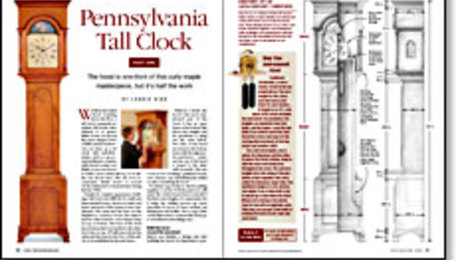This image appears to be a two-page color magazine ad for the Pennsylvania Tall Clock. The left page prominently features a tall, slender, oak-colored grandfather clock that occupies the vertical length of the page. Beside this clock, the title "Pennsylvania Tall Clock" is written in large red font, and beneath it lies an article, the text of which is detailed but unreadable. Centrally placed within the page is a photograph of a person wearing a black shirt, seemingly engaged in adjusting the clock, possibly setting the time. The right page continues with a column of red text on the left, which appears to describe a series of black and white diagrams. These diagrams depict various views and the internal mechanisms of the Pennsylvania Tall Clock, revealing the intricate details and craftsmanship of the timepiece.